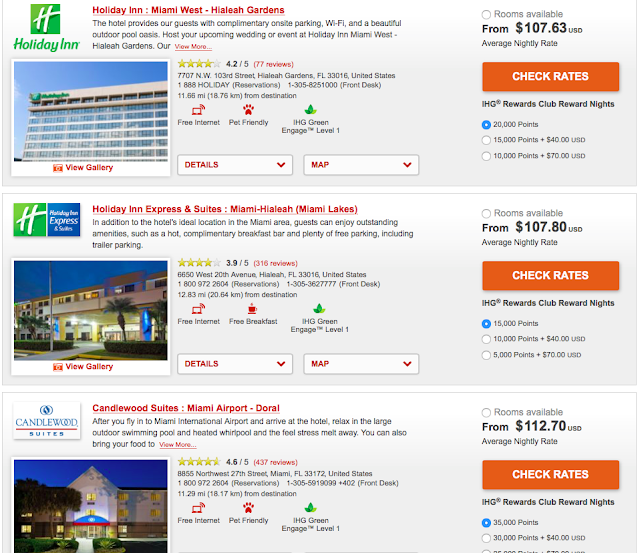In the image, someone seems to be searching for hotel stays, likely in the Miami area. The interface showcases three rectangular advertisement boxes promoting hotel accommodations. 

The first box highlights the "Holiday Inn Miami West, Hialeah Gardens." The advertisement features a distinctive green box with an "H" symbolizing the Holiday Inn brand. The accompanying text reads, "Holiday Inn Miami West, Hialeah Gardens: The hotel provides guests with complimentary on-site parking, Wi-Fi, and a beautiful outdoor pool oasis. Host your upcoming wedding or event at Holiday Inn Miami West, Hialeah Gardens." 

Displayed on the right side of the box is an orange button labeled "Check Rates" in white text. The average nightly rate starts at $107.63 USD. Additional icons denote amenities including "Free Internet," "Pet Friendly," "IHG Rewards," and "Green Engage Level 1" certification. 

A thumbnail image of the hotel's exterior appears on the left, with an option to "View Gallery" for more photos.